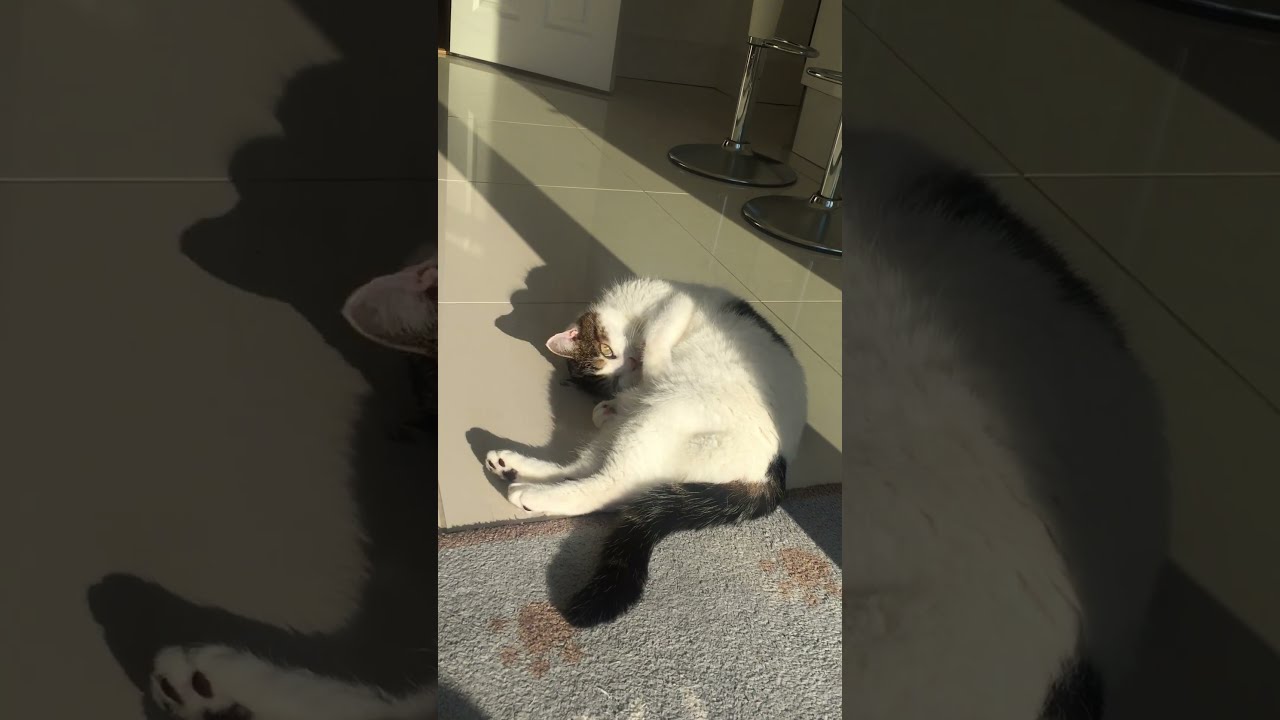This is a photograph of a very cute and very fat white short-haired calico cat with small black spots, lounging on a tiled patio in the sunshine. The image is in portrait orientation, a vertical rectangle, with the cat laying in the center of the frame. The majority of the cat's body is illuminated by the sunlight, casting long shadows across the tiles, while part of its upper back lies in the shadow of a nearby pole. The cat is laying on its right side with its front paws bent upward towards its chin, appearing relaxed and likely asleep, while its hind legs are in a comfortable position—the left slightly extended and the right tucked in towards its belly. The cat's face and tail are not visible in the image. In the foreground, right next to the cat’s lower body, is a gray and brown carpet with a brown trim. Behind the cat, towards the top of the image, there's the wall of a house and what appears to be a door, with the bases of some stools visible on the right side. The colors in the image include shades of black, white, gray, beige, and silver. This charming scene, especially captivating for cat lovers, captures the serene moment of the cat basking in its sunny spot.